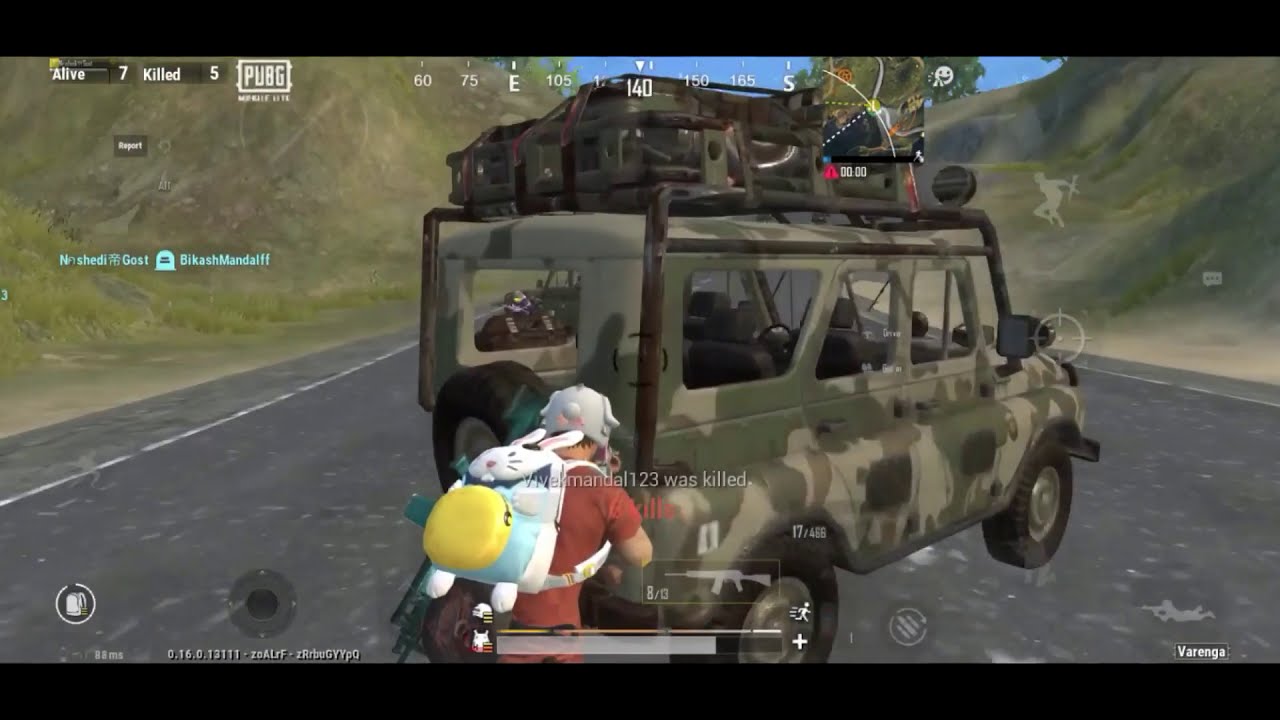The image is a detailed screenshot from the video game PUBG. It features a military jeep parked sideways in the center, facing away to the right, showcasing a half-right profile with visible right-hand side and rear. The jeep is painted in camouflage and loaded with equipment on the top rack. Behind the jeep, a person in a red t-shirt, white cap, and white backpack, with a yellow canister attached, walks away from the viewer. The person is positioned near the back right-hand side of the vehicle. The scene is set on an asphalt road stretching into the distance, flanked by greenish hills on both the left and right sides. The top of the image shows a patch of blue sky. Various in-game elements frame the scene, including the text "alive" and "killed" in the upper left corner, and compass readings along the top center. The colors in the image range widely, featuring different shades of green, white, gray, red, yellow, light blue, pink, brown, and tan.